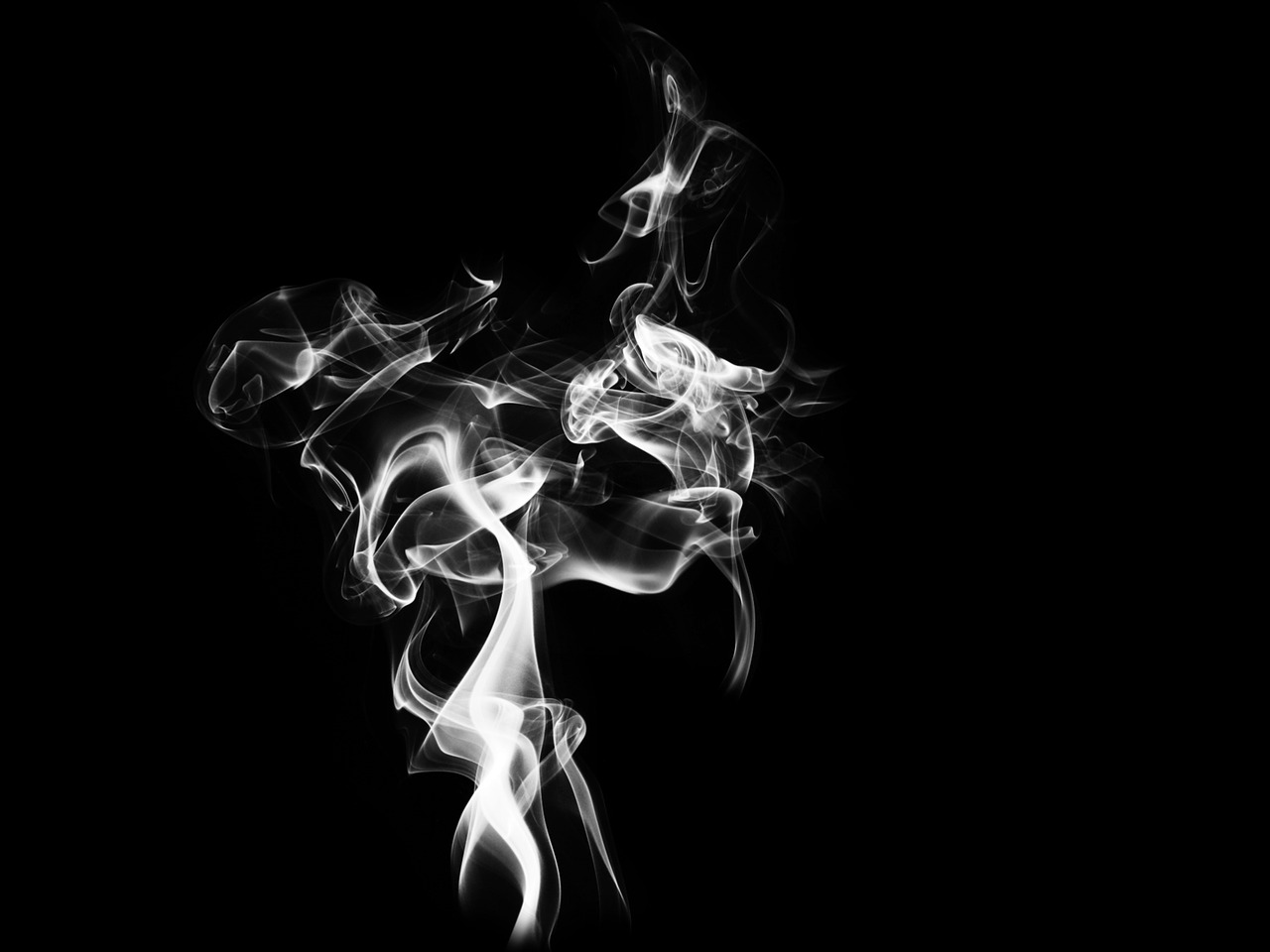This black and white art piece presents an intricate display of smoke rising from the bottom to the top of a completely black background. The smoke, rendered in shades of grayish-white, begins thicker at the base and thins out as it ascends, creating a variety of unique, swirling patterns. As it moves upwards, it becomes translucent in spots, with lines crossing over each other and delicate loops and puffs forming. The smoke’s trajectory is random, with some wisps moving all the way to the top, some flowing off to the sides, and others forming tiny streams that connect back to the main body. This slow-motion effect evokes a sense of lingering motion. The abstract nature of the piece invites personal interpretation; one viewer might see a sports figure holding a trophy, while another might discern a tree-like structure with its branches spreading out. Every viewer is encouraged to find their own meaning within the flowing, ethereal forms.